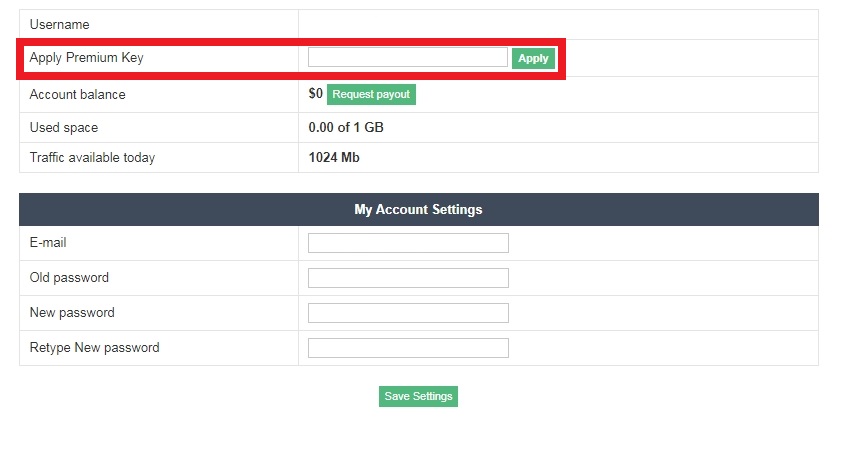The image displays a user interface in a rectangular box segmented into five rows and two columns. The first row contains a field labeled "Username," and the second row hosts a field titled "Apple Premium Key." This field is encircled by a thick, solid red line, indicating its importance or required input. Users can type into this field. Adjacent to it is a prominent green button labeled "Apply."

Beneath this section, the following account details are presented:
- "Account Balance," displayed as 0,
- "Requested Payout,"
- "Used Space," showing 0.0001 gigabytes,
- "Traffic Available Today," listed as 1024 MB.

An open white space follows these details.

Below the white space is a blue bar adorned with white text that reads "My Account Settings." In this section:
- The field labeled "Email" is housed within a square rectangle,
- The "Old Password" and "New Password" fields are also boxed,
- The "Re-type Password" field is included as well.

At the bottom of the settings section is a green button, with "Save Settings" written in white text, ready to finalize any changes made.

This comprehensive layout is designed to facilitate straightforward management of user account details and settings.